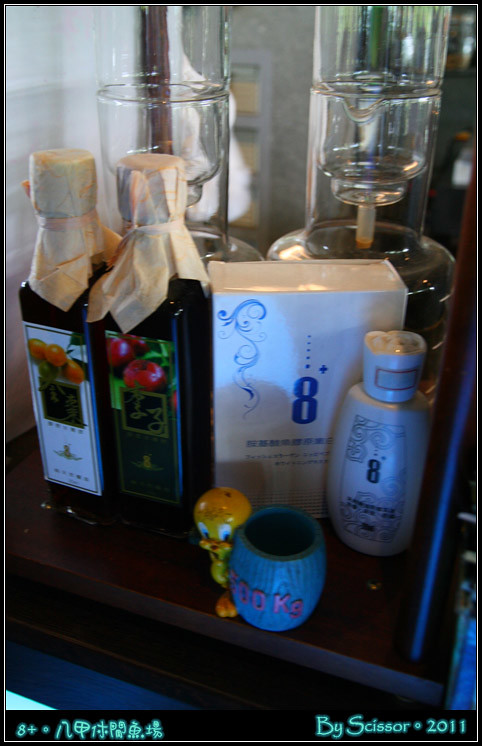The image appears to be a detailed and thoughtfully arranged photograph or poster showcasing a small bar setup. At the bottom right corner, there is a signature that reads "By Scissor 2011." On the bottom left, there are characters, likely in an Asian script, whose meaning is unclear.

The poster is enclosed in a thin black frame. The scene inside features multiple layers and intriguing items. On the left side, there’s a white door leading to another room framed in brown. In the forefront is a black tabletop cart. Prominently displayed on the cart is a small blue barrel mug or cup, next to which stands a Tweety Bird figurine, colored in yellow, blue, orange, and red.

Next to the Tweety Bird, there is a distinct white bottle and a matching white box, both marked with the number 8 in blue. Beside these are two square dark bottles, one adorned with a label depicting red cherries with green leaves, and another showing an orange fruit, perhaps apricots or oranges, also with green leaves. These labels feature elegant designs with gold and black highlights. The bottle tops are covered with a cream-colored paper or fabric, tied with string.

In the background, slightly obscured, stand several large glass containers that resemble decanters. These could serve a specialized function, such as distilling or filtering, adding to the sophistication of the display. The overall setup has a reflective quality, likely due to a mirrored back, enhancing the visual depth of the arrangement.